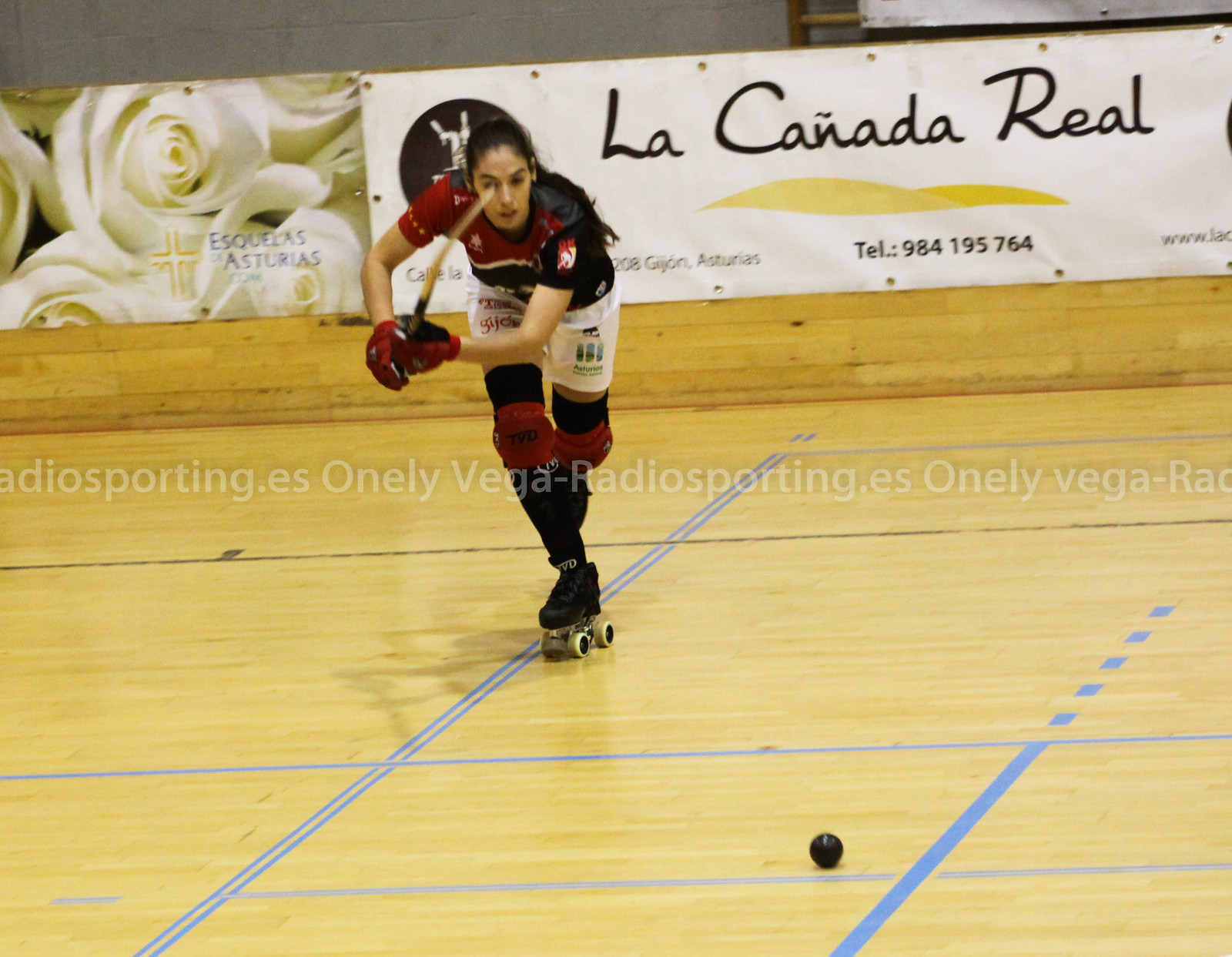A young woman with long black hair tied in a ponytail is captured indoors in a gym, playing a sport that resembles indoor hockey. She is equipped with roller skates that have two wheels in the front and two in the back. She dons black and red knee pads, white shorts, long black socks, and a black and red jersey. Her stance is dynamic, with one foot extended forward and her arms raised, gripping what appears to be a hockey stick. The gym floor features blue grids laid out diagonally and horizontally, with a round black ball positioned within one of the squares. Behind her, a white sign with black text reads "La Canada Rio." Additionally, the background includes elements such as shapes and perhaps astrals with white roses, and there’s a visible watermark at the center of the image that reads "Onelivega-radiosporting.es."